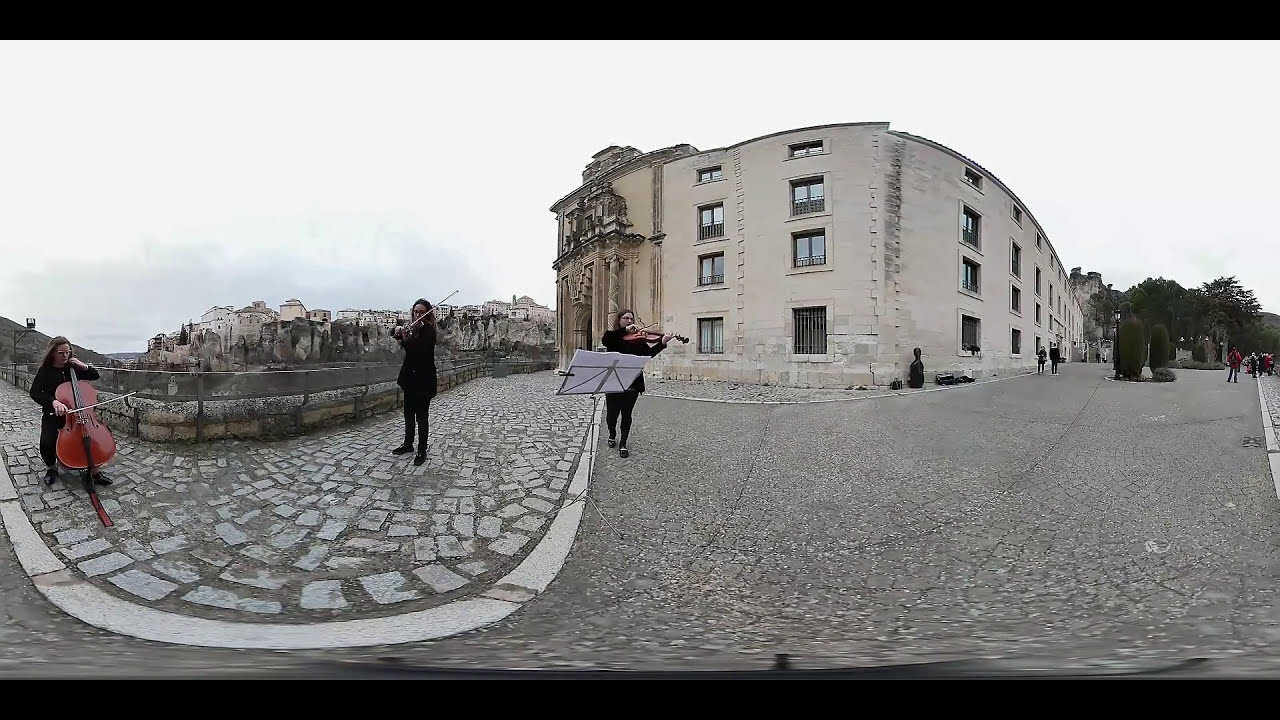This photorealistic image depicts a cloudy outdoor scene dominated by a large, ornate light gray brick building with an intricately carved entrance. The building spans multiple windows, some adorned with bars, and features decorative architectural elements extending around its three to four stories. The ground is a cobbled gray stone, interspersed on the left side with white stones forming a patterned path.

In the center of the image stands a lady dressed in black with long hair, playing a brown violin. In front of her is a music stand with white pages. To her left, another woman in black is also playing a violin, and further to the left, another lady, also in black and sitting down, is playing a larger brown-red string instrument, likely a cello.

The background reveals a fenced-off barrier and a large dip or valley, beyond which a village of white and light brown buildings rises over steep gray cliffs. To the right, darker gray trees are visible in the distance, with crowds of people closer to them. The sky is a light white with patches of light gray towards the horizon on the left. The overall scene is punctuated with various people walking around, contributing to the bustling ambiance of this picturesque, historic setting.